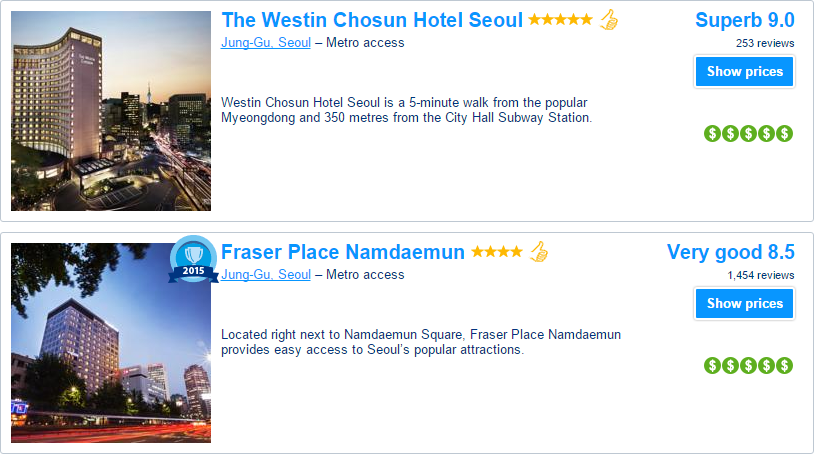This image from a travel website showcases two hotel listings. 

The first listing features the Westin Chosun Hotel in Seoul. Displayed prominently is a photo of the hotel building. The hotel boasts a five-star rating, indicated by five stars and a thumbs-up icon labeled "Superb" with a rating of 9.0. The location "Janggu, Seoul" is highlighted in blue and underlined, indicating a link, followed by a note on its convenient "Metro Access." A button on the right prompts users to "Show prices." 

Below the image are details about the hotel's prime location: "Westin Chosun Hotel, Seoul. It's a five-minute walk from the popular Myeongdong and 350 meters from the City Hall subway station." Additionally, five green circles with dollar bills point to the pricing tier.

The second listing is for Fraser Place Namdaemun, also featuring a photo of the building. It highlights an award icon for 2015, located in Janggu, Seoul, with "Metro Access" noted. The hotel has an impressive rating of 8.5 based on 1,454 reviews. This listing follows the same format as the first, providing consistent and easy-to-read information for the user.